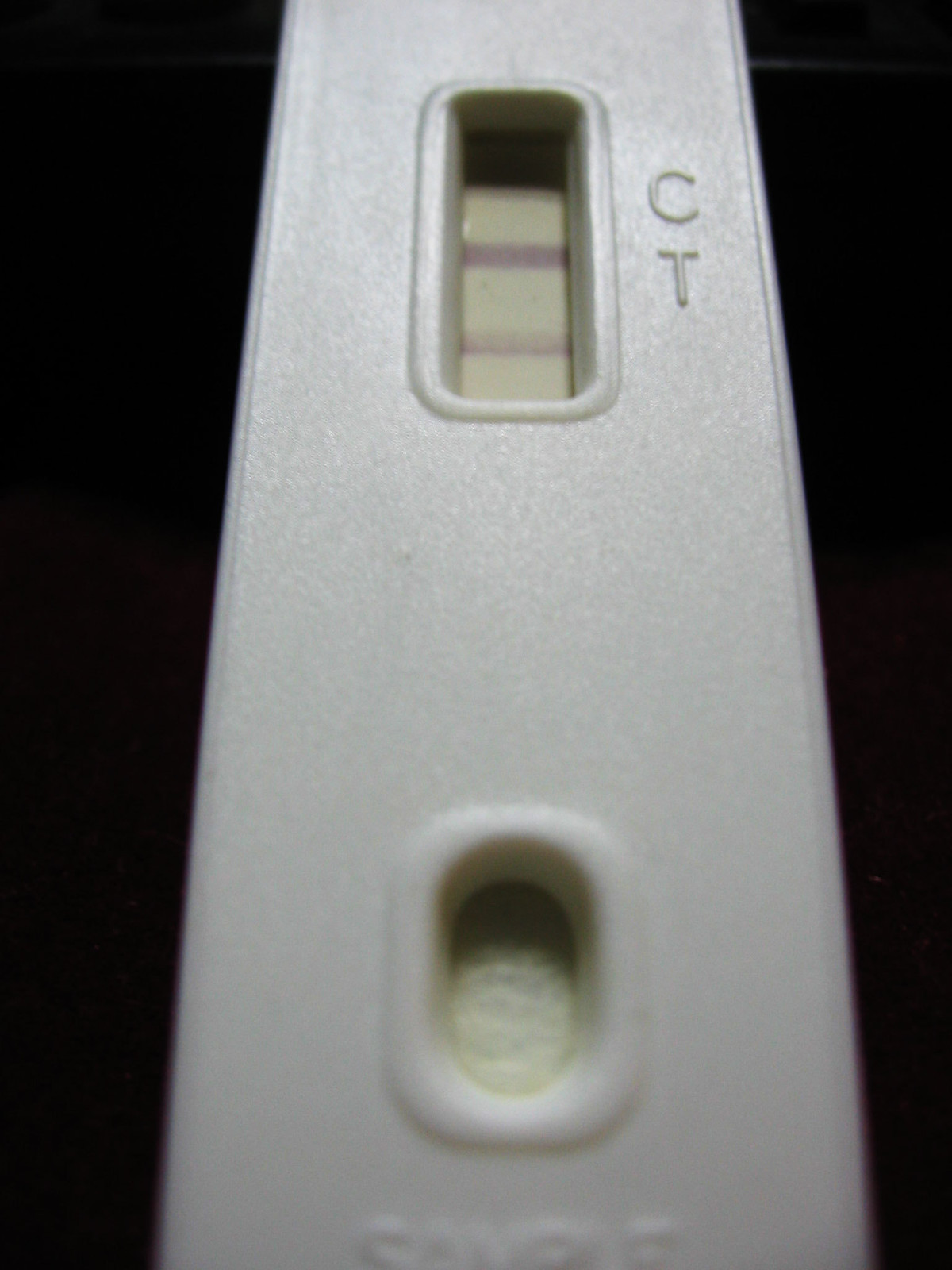This image showcases a close-up view of a test strip, which could be for a pregnancy test, a COVID test, or a drug test. The background is entirely solid black, with a subtle light spot visible in the top right corner, barely noticeable through the dark expanse. The test strip itself is a white plastic stick, extending from the top to the bottom of the photograph, with both ends cut off by the frame. The stick is leaning slightly, making the top appear narrower than the bottom.

In the middle of the test strip, there is a small rectangular window displaying a white piece of paper with two distinct pink lines. Adjacent to this window, the characters 'C' and 'T' are printed, indicating the control and test lines. Below this window, another oval-shaped opening contains a piece of cotton, likely used for sample collection or application. Further down, the word "SAMPLE" is raised in the plastic, marking the spot where the sample should be applied. The overall focus is on the intricate details of the test strip against the stark contrast of the black background.